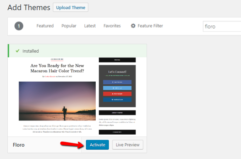The image depicts a blurry screenshot of a webpage set against a light gray background. At the top, there's a navigation bar alongside a search bar positioned at the top right corner. Below, the main content area features a striking image of a man standing on a beach, his back silhouetted against a vivid sunset with hues of orange and blue painting the sky as the sun dips below the horizon. The man gazes out contemplatively towards the sea. The webpage includes a message that reads, "Are you ready for the new..." followed by indistinct text. Various buttons are scattered throughout the page, one of which has an arrow pointing towards it, starting with the letter 'A'. The content also mentions options to "add themes" and includes an "upload theme" button, suggesting customization features likely related to web design or theme creation.